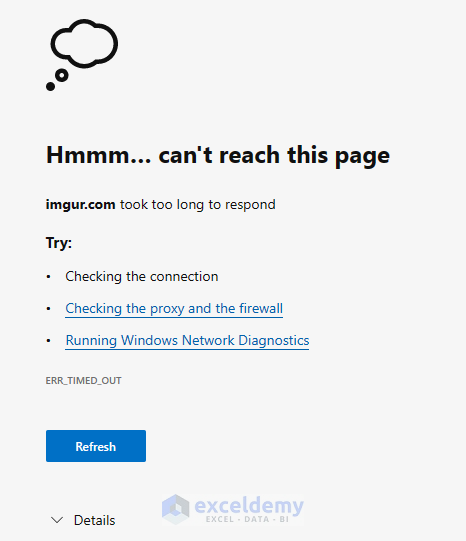The image depicts a Microsoft Edge browser window displaying an error message indicating that the page could not be reached. The message, "Hmm, we can't reach this page," is accompanied by a thought cloud icon above it. The URL "imager.com" failed to load due to a timeout error, specifically "ERR_TIMED_OUT." The error message suggests several troubleshooting steps: checking the internet connection, examining proxy and firewall settings, and running Windows Network Diagnostics. At the bottom of the error message, there is a refresh button and a "Details" drop-down arrow for further information. Additionally, there is a watermark in the bottom right corner that reads "Excel Demi," likely the logo or identifier of whoever captured the screenshot. The watermark notes that either the imager.com website was not working at the time or the user’s internet connection was experiencing issues. The user appears to have been testing Microsoft Edge, possibly to check website functionality across different browsers.